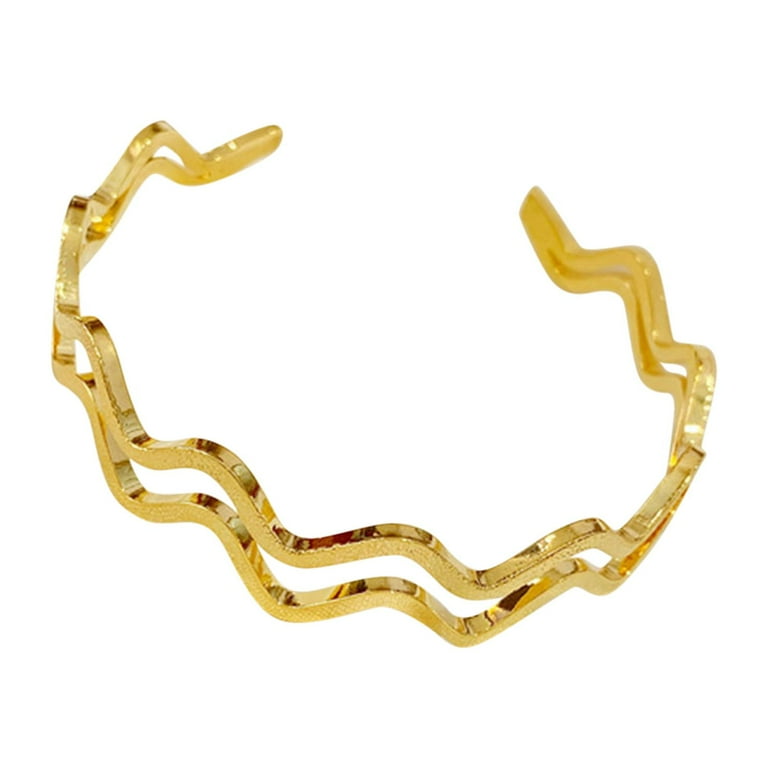The image depicts a shiny, gold bangle bracelet set against a white background. The bracelet, characterized by its open-ended, semi-circular design, features two wavy, zigzag-patterned strands of gold that create a visually striking effect. These intertwined, undulating lines give the impression of embedded diamonds due to the intricate cuts and high polish. The overall appearance is one of sophistication, with the alternating peaks and valleys of the zigzag pattern adding depth and texture. The bracelet lacks a clasp, suggesting it’s designed to be easily slipped onto the wrist. The vibrant gold and shimmering finish make the bracelet eye-catching and elegant.